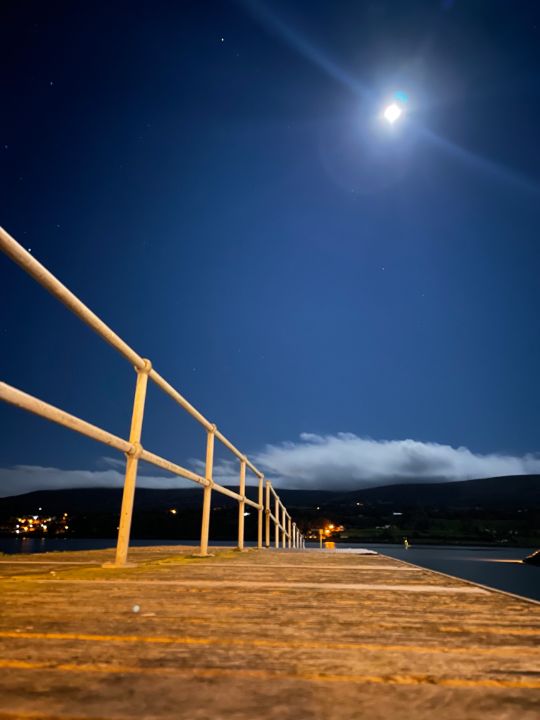In this evocative evening scene, a solitary wooden pier stretches out over a calm body of water, possibly a river or lake, under a mesmerizing night sky. The sky transitions from a deep black at the top to a gradient of blues, culminating in lighter hues and white clouds above a dark mountain range. To the right, a glowing full moon adorns the sky, adding to the serene ambiance. Distant white lights from buildings sprinkle the horizon beneath the mountains, suggesting a distant town or cityscape. The pier, featuring a prominent yellow metal railing in the middle, leads the viewer's eye towards the tranquil water, with no people or animals in sight. The photo captures a peaceful, almost mystical moment, blending natural beauty with tranquil human footprints, in a scene where the dark blue water and the black silhouette of the hills enhance the overall mystique.